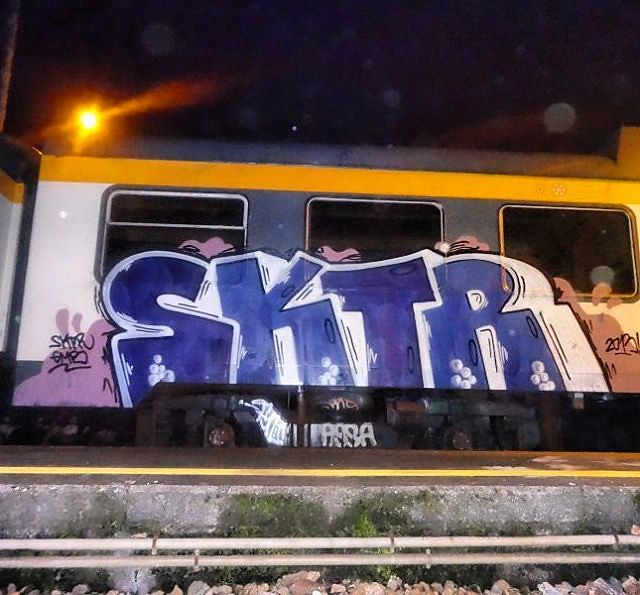In this evocative image, we see an abandoned train or subway car sitting above concrete slabs and gravel-strewn railroad tracks. The scene captures a dark, almost dusky atmosphere with faint sunlight peeking through the left side, contrasting with the illuminated streetlight in the background. Dominating the side of the train is bold graffiti lettering spelling "SKTR" in large, block-like blue letters with a distinctive white outline and various white dashes and bubbles. There's also additional graffiti on the left side, smaller black initials, potentially "GMR," with an ambiguous sequence, and another part possibly reading "20p." The train car itself is adorned with a yellow stripe at the top and is primarily white with gray trim. Below the graffiti, you can make out several lines resembling the bottom of the train car or subway. Further details include three windows above the graffiti, although it's difficult to discern any interior details due to the darkness. The overall graphic appearance suggests a blend of urban decay and artistic expression.